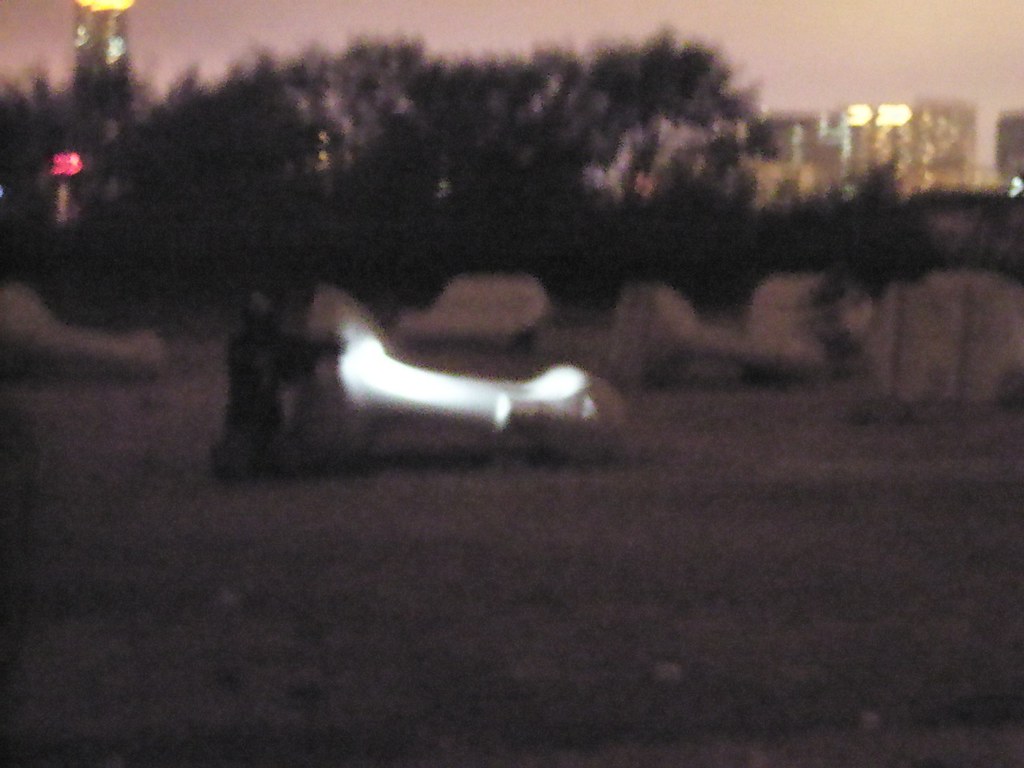In an evening outdoor setting, a person, possibly a man dressed in a hoodie and jeans, is kneeling on the pavement beside a road. He is interacting with a large, enigmatic metal object on the ground, which appears too substantial to be a simple car part. Scattered around the object are various other items that seem to have fallen. Behind him, the scene is framed by trees, while to the far right, a tall, illuminated building stands prominently.